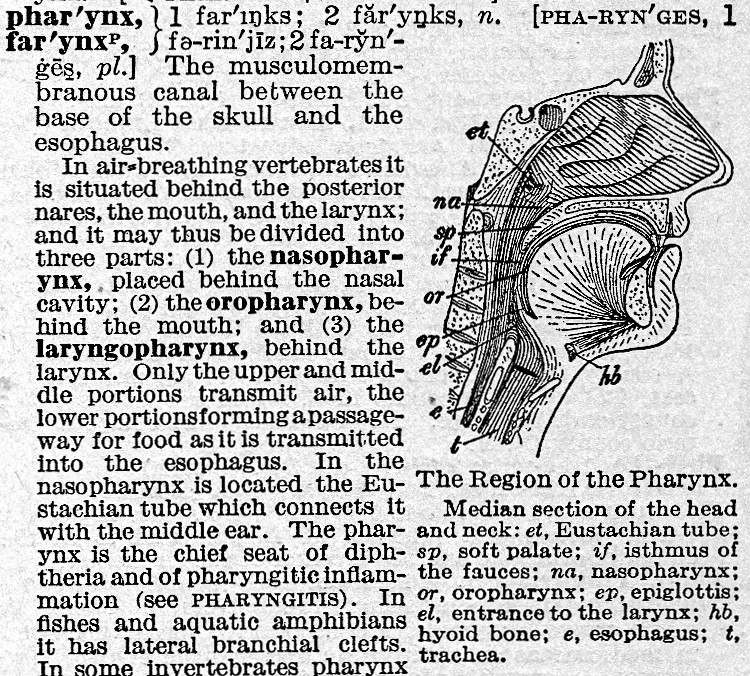This image, likely an excerpt from a medical or physiology textbook, provides a detailed definition and anatomical description of the pharynx. The left-hand column begins with various pronunciations of the word "pharynx" and defines the pharynx as a musculomembranous canal extending between the base of the skull and the esophagus. It explains that in air-breathing vertebrates, the pharynx is located behind the nasal passages, mouth, and larynx, and divides into three regions: 1) the nasopharynx behind the nasal cavity, 2) the oropharynx behind the mouth, and 3) the laryngopharynx behind the larynx. The upper and middle portions allow air passage, while the lower portion serves as a food conduit to the esophagus. The nasopharynx houses the Eustachian tube, which connects to the middle ear. Additionally, the pharynx is identified as the main site for diphtheria and pharyngitic inflammation (see pharyngitis). In aquatic species, such as fishes and amphibians, the pharynx features lateral brachial clefts. Some sections of the text are cut off mid-sentence.

On the right side of the image is a sketched, grayscale anatomical diagram of the pharynx, including labeled parts of the head and neck. The labels correspond to various structures, including ET (Eustachian tube), SP (soft palate), IF (isthmus of the fauces), NA (nasopharynx), OR (oropharynx), EEP (epiglottis), EL (entrance to the larynx), HB (hyoid bone), E (esophagus), and T (trachea). Below the illustration, additional text offers a median section view of the head and neck, listing these anatomical features. The background of the page is gray, and the text is printed in black, arranged in two columns, providing a comprehensive overview of the pharyngeal region.